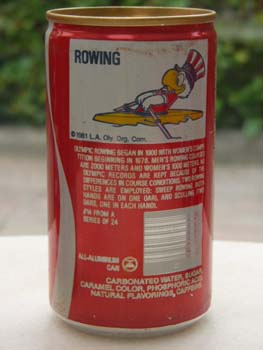This image features a red soda can, presumably a Diet Coke, as suggested by its distinctive design elements. The can is characterized by a brass-colored top and a familiar silver stripe of varying width running vertically along its surface. The view depicted is from the back of the can, where a UPC code and other ingredient details are prominently displayed. At the top of the can, a white rectangular label contains a square graphic of an eagle wearing an Uncle Sam hat and rowing, possibly part of the branding or a promotional event. The text beside the graphic reads "Copyright 1981," followed by "L.A. something," which is partially obscured.